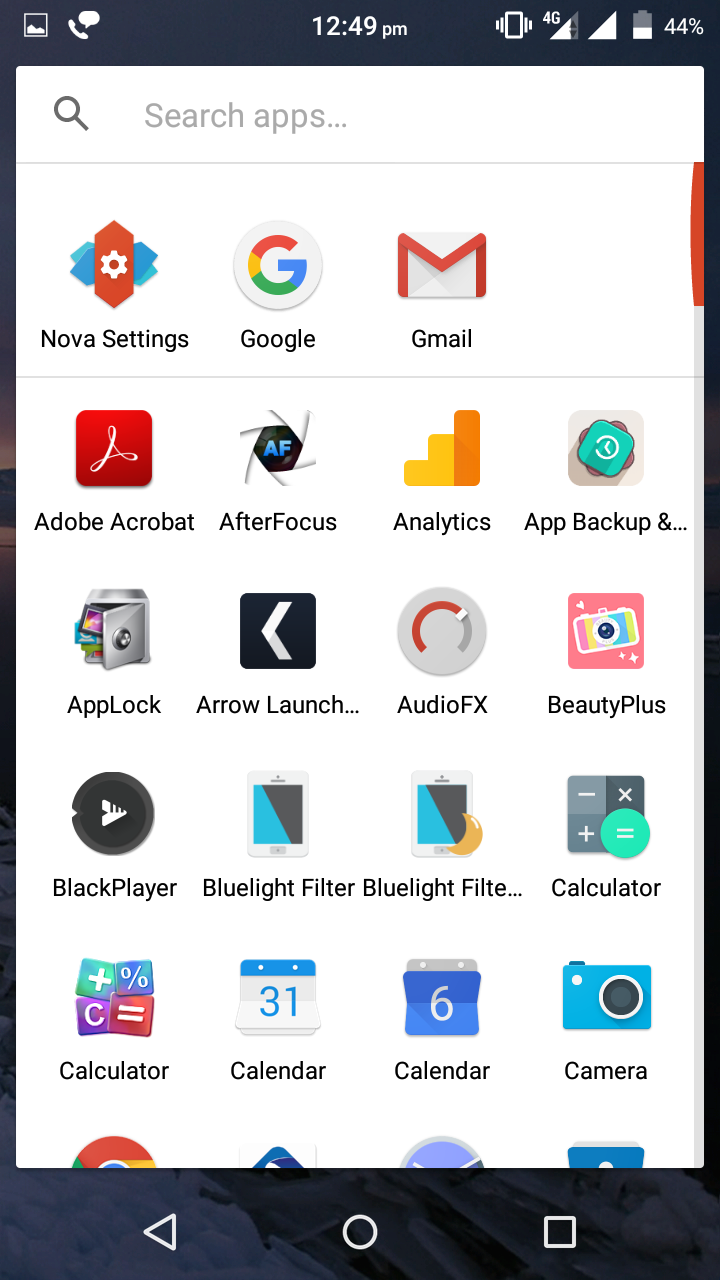A smartphone screen displays the current time at the top center as 12:49 PM. The device is connected to a 4G network with 44% battery remaining. The user has accessed the ‘Search Apps’ feature, displayed prominently below the status bar. The topmost row of icons includes Nova Settings, Google, and Gmail. These icons are separated by a fine gray line from the next set of applications below. The lower section contains various app icons: Adobe Acrobat, After Focus, Analytics, App Backups, an indistinct icon, App Lock, Arrow Launcher, Audio FX, Beauty+, Black Player, Blue Light Filter, another Blue Light Filter with a moon symbol, Calculator, another Calculator with a different icon, Calendar, another Calendar with a different icon, Camera, Chrome, and three additional icons partially obscured, requiring scrolling to be fully viewed. Recognizable icons like Chrome and Adobe Acrobat are among the visible apps, indicating commonly used functionalities.